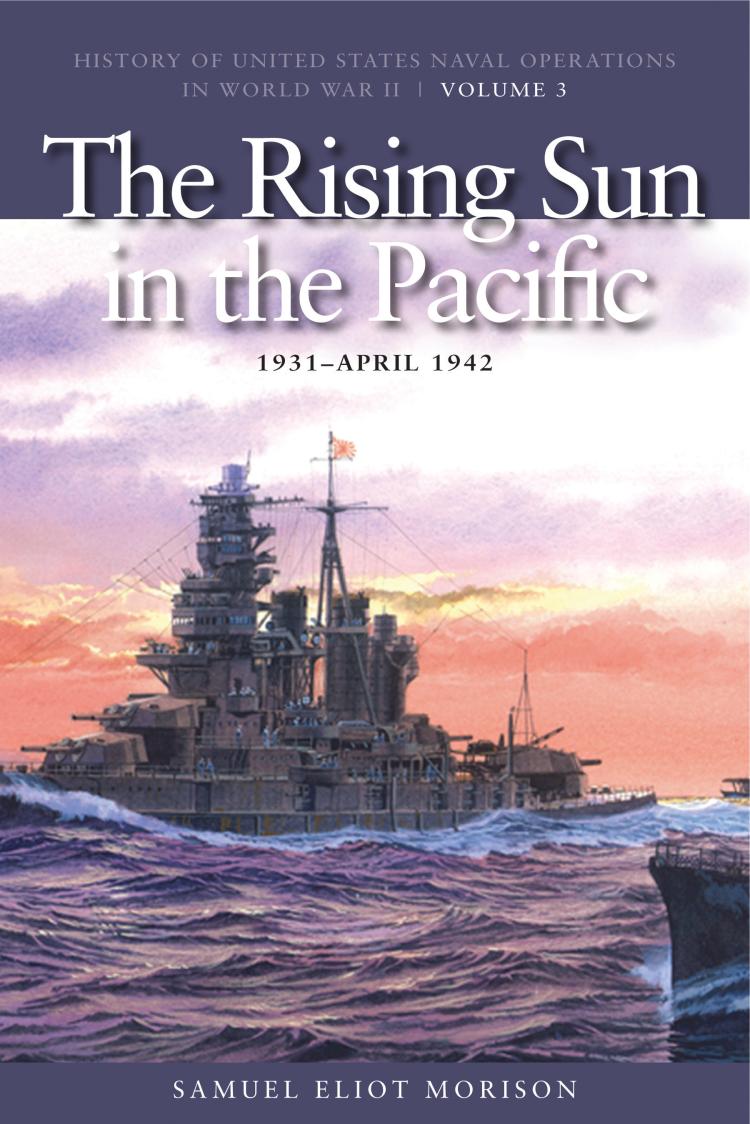The image is a cover of a book titled "The Rising Sun in the Pacific, 1931 to April 1942," authored by Samuel Elliott Morrison. This is the third volume in the series "History of United States Naval Operations in World War II." The cover features a detailed depiction of a large gray battleship, possibly a destroyer, bristling with numerous gun turrets and multi-story towers equipped with various radio communication equipment. The ship navigates through rough, choppy, purplish water with waves crashing over it. Above the battleship, the sky transitions from pink at the horizon, suggesting a sunrise or sunset, to layers of white and purple clouds. The top of the cover displays a dark blue rectangle with the title and dates in large white and black letters. The entire image evokes a scene of naval warfare set against a dramatic sky and turbulent sea.